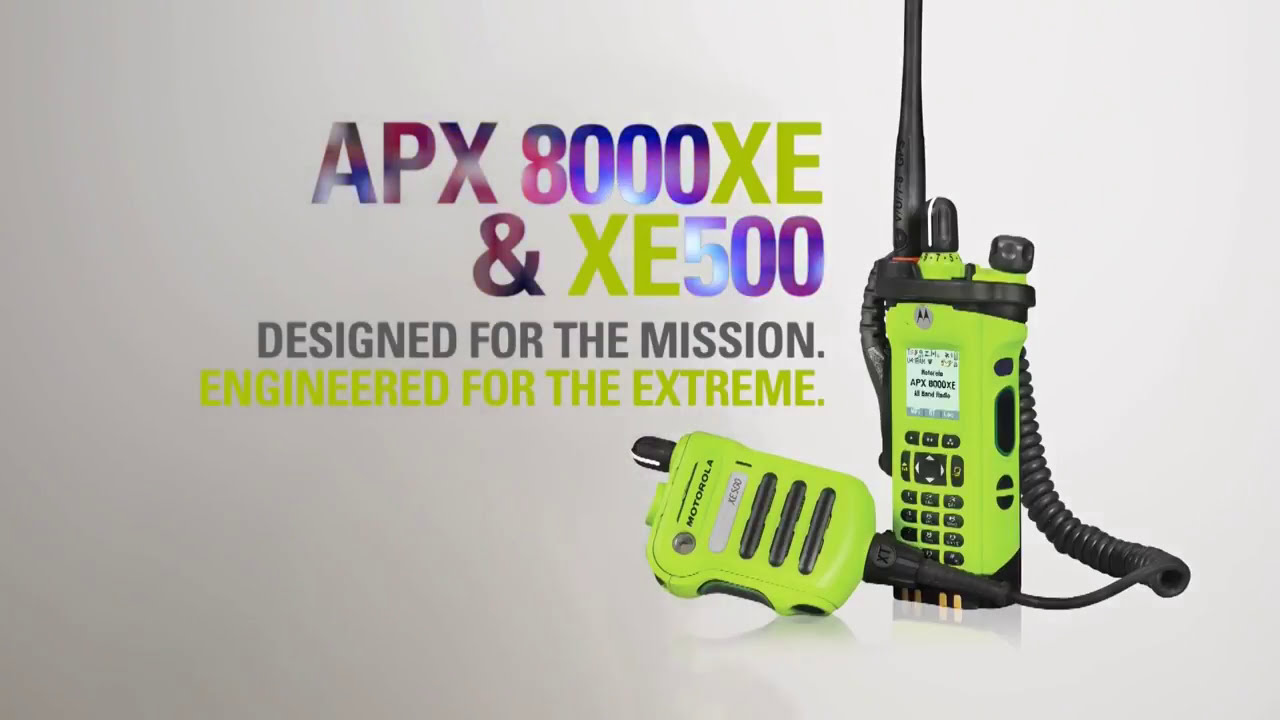The advertisement showcases a bright lime green portable radio, resembling an old "brick" mobile cell phone, set against a gray gradient background transitioning from dark gray on the left to light gray on the right. This Motorola APX-8000XE radio, engineered for extreme conditions and designed for mission-critical use, features a tall black antenna, black buttons, and black cords. The attached handheld mic enhances its functionality. Prominent text at the upper left corner of the image reads, "APX-8000XE and XE-500," followed by the tagline, "Designed for the mission. Engineered for the extreme," emphasizing the product’s durability and innovative design.